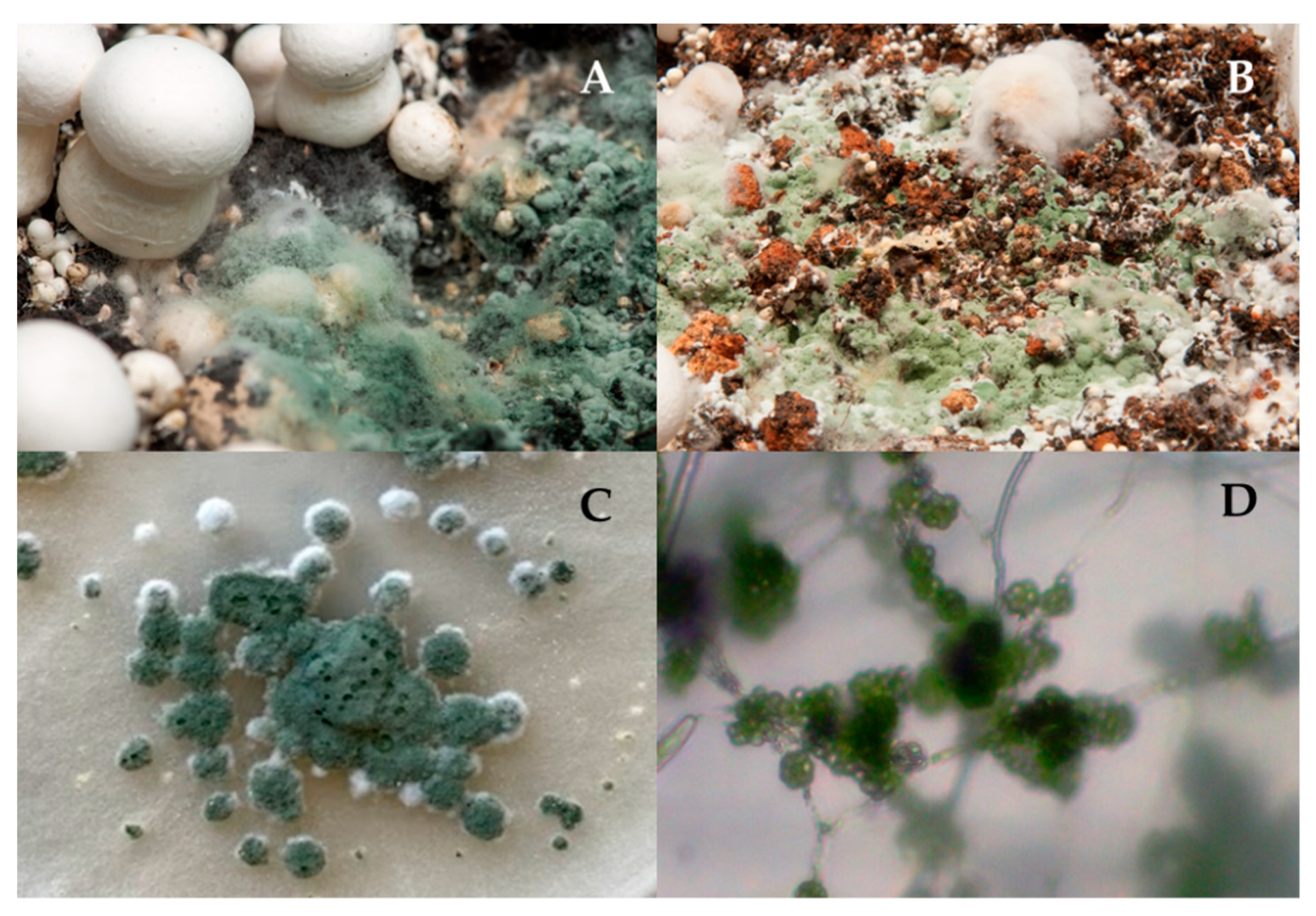This image is a collage of four microscopic photographs arranged in quadrants labeled A, B, C, and D, in a square pattern. Each photograph provides a detailed view of various fungal or mold growths, all with a distinctive bluish-green hue suggestive of fungal spores or mold. 

In quadrant A, the image depicts what appears to be mushroom spores. These are characterized by a bluish coloration akin to moldy cheese, surrounded by white structures that resemble macaroon cookies or button mushrooms. Quadrant B, a similar image, includes not only bluish spores but also some reddish spores, enhancing the complexity of the observed fungal structures.

Quadrant C, located below A, presents an even more magnified view with a white background and dark green, bumpy formations that also have patches of white. Finally, quadrant D shows features on a white background with a greenish, molecular-like texture. This section appears somewhat blurry and has been described as resembling small bobas or spheres, indicating intricate fungal or mold patterns.

Overall, the collage offers a detailed exploration of fungal spores or mold microorganisms under high magnification, with variations in coloration and structure across the different quadrants.